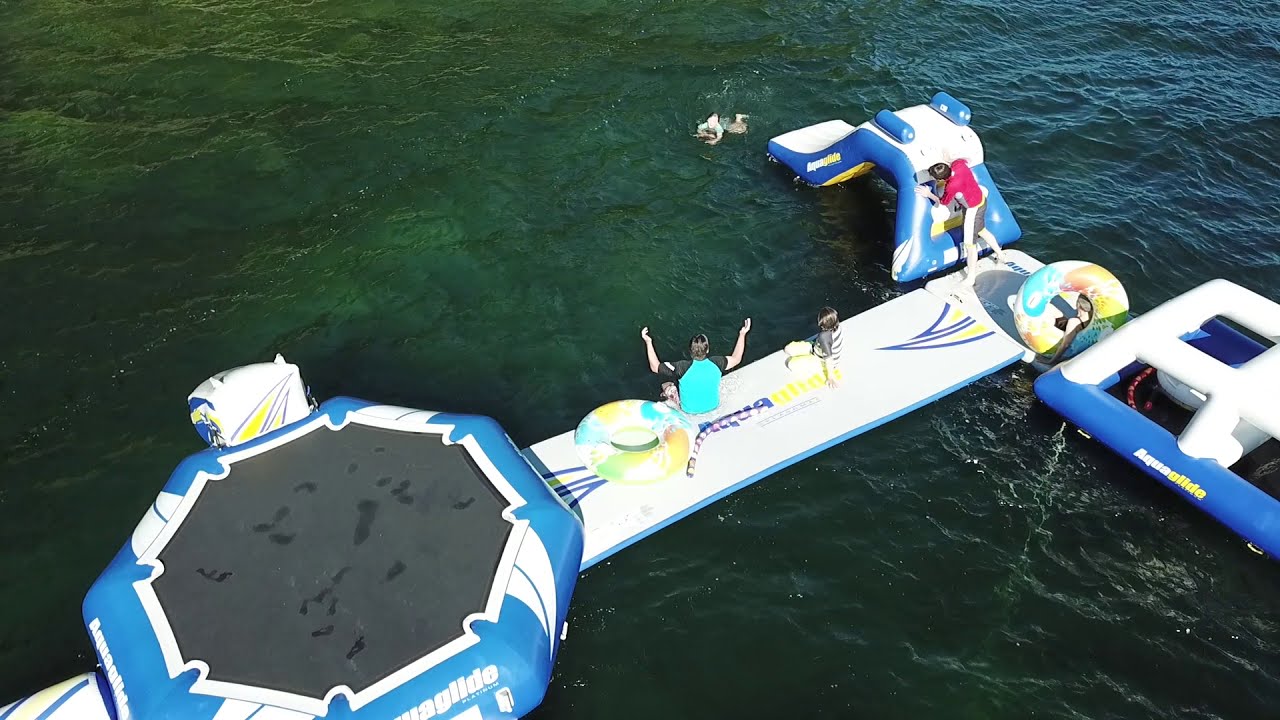This daytime aerial photograph captures an outdoor recreational scene set in open waters, where a variety of inflatable play structures float. Dominating the lower left corner is an octagonal trampoline featuring a black tarp and blue-and-white inflatable borders. Visible on the trampoline are dark footprints, suggesting recent use. Extending from the trampoline toward the upper right, the interconnected structures include a circular donut-style ring and a slide. A man of Caucasian descent, dressed in a blue and black short-sleeved water top, raises his arms as he sits with his children on the inflatable raft. In the upper right-hand area of the image, another adult wearing a red top stands at the back of the slide, watching a child who has just splashed into the water. The water itself transitions from a green hue on the left side of the photograph to a deeper blue in the upper right corner, creating a vibrant backdrop for this floating activity center. Scattered text on some inflatables reads "Aqua Slide" or "Aqua Glide," although it remains somewhat blurry. This vivid scene showcases various colors encompassing green, blue, black, white, red, yellow, gray, and orange, with the focus on the playful inflatables at the center of the image.